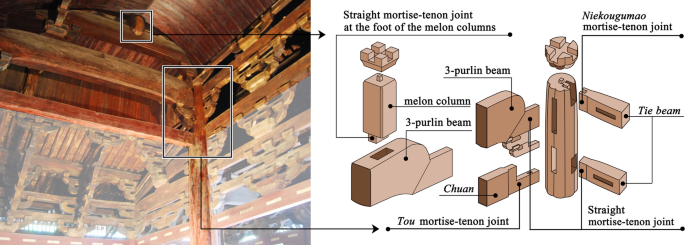The image showcases a detailed instructional graphic depicting the assembly of a wooden interior roof structure. On the left, a color photograph illustrates the completed ceiling section, featuring a view looking up into the intricately joined woodwork. This photograph includes two rectangular blowout sections outlined in white, each pointing to specific areas of interest within the ceiling. On the right side, an accompanying illustration provides a breakdown of the individual wooden components and their connections, highlighting various wooden shapes and how they interlock through mortise and tenon joints. The text over the top reads "Straight Mortise-Tenon Joint at the Foot of the Melon Columns," with additional labels such as "melon column," "three purlin beam," and "tai beam" annotating each part. The illustration employs a blend of photographic realism and graphic design to clearly represent the detailed craftsmanship involved in constructing the wooden ceiling.